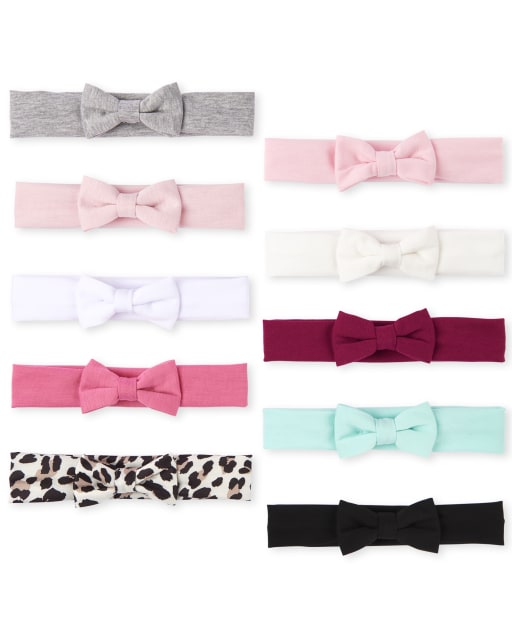This image displays a collection of 10 small bow-style headbands, likely designed for a baby or toddler, arranged on a flat, white background. The headbands appear to be composed of nylon and are conveniently designed to stretch over the head. On the left column, from top to bottom, there is a gray bow headband, followed by a pink one, a very light purple bow bordering on white, another pink bow, and a cheetah print bow. The right column, from top to bottom, features a light pink bow, a white bow, a maroon bow, a teal or mint green bow, and finally, a black bow. Each headband has a bow positioned at the center, ready to adorn a little girl’s hair.